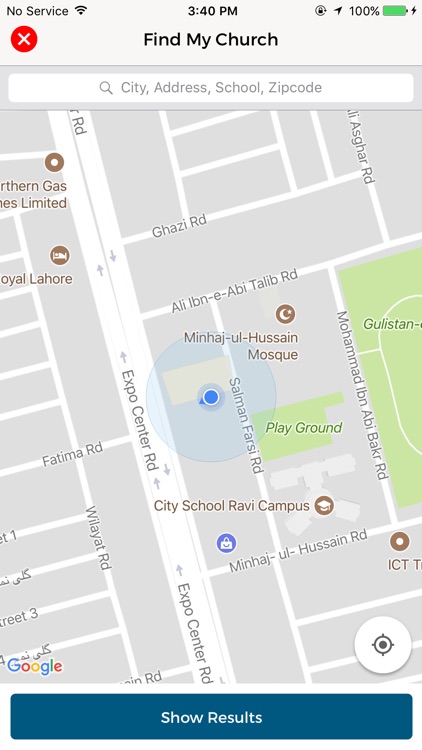This image, captured on a cell phone, showcases the "Find My Church" application. At the top of the screen, there's a navigational circle containing a white 'X', allowing users to dismiss or exit the app. The main portion of the display features a detailed map highlighting various landmarks, including Fatima Road, Mahi Hassan Mosque, City School Rabi Campus, Ghazi Road, Northern Gas Southern Limits, and Royal Lahore.

Additionally, a green area designated as a playground is visible near the school. The map has a radar-like emanation marking the user's location, surrounded by brown circles with white icons that illustrate different points of interest. One such icon resembles a graduation cap, indicating the presence of a school. At the bottom of the interface, there's a prominent deep teal button labeled "Show Results", which users can press to retrieve search findings related to their query for churches.